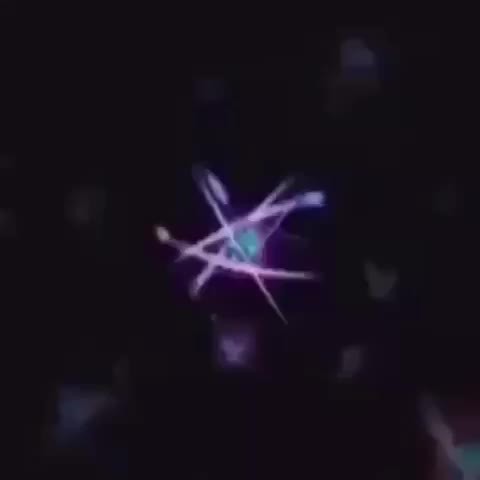The image is a muted, square-shaped graphic or low-resolution photograph, characterized by its very dark, almost black background. At the center, a blurred, round blue-green orb is visible, surrounded by several circular, colored light trails. These trails vary in color, appearing purplish-pink or lighter shades, resembling motion trails or energy paths. The light trails and orbs create a star-like formation, somewhat akin to electrons or particles orbiting a nucleus. Additionally, scattered throughout the dark background are smaller, less distinct light spots, contributing to the overall impression of a distant star or constellation in the night sky.